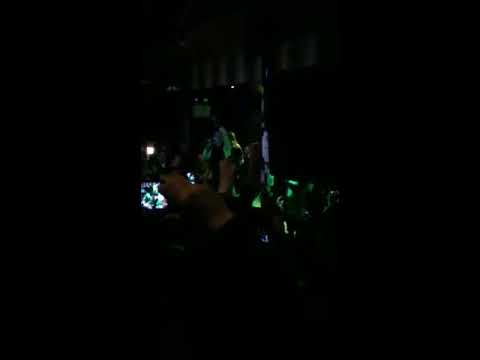The image is a small square with a predominantly solid black background. At the very center, the scene is dimly lit and somewhat blurry, making it difficult to discern specific details. There appears to be a faint combination of brown, green, and a touch of purple, suggesting the presence of illuminated subjects in an otherwise dark setting. One can barely make out what seems to be a scene involving people—potentially an audience at a show or concert—where a green light casts a glow on their bodies. In this central area, a brown object that might be a curtain hangs down at the top, suggesting an indoor setting. On the left side, there is a faintly visible arm holding a lit-up phone, possibly capturing the moment. The lack of clarity and the overwhelming darkness contribute to the difficulty in identifying the exact nature of the scene.